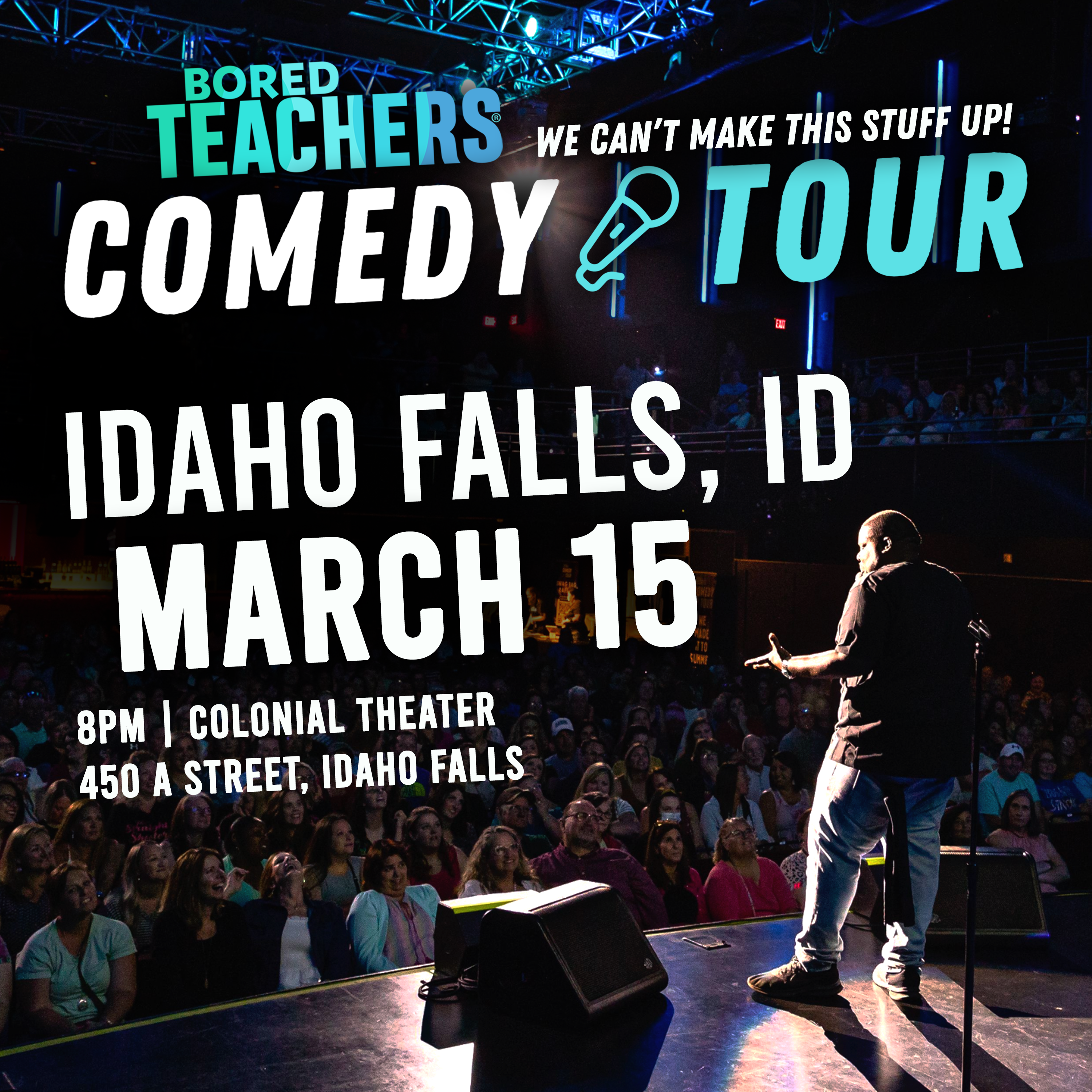This image is an advertisement designed in portrait orientation, depicting a man on a stage in front of a packed audience. The setting is a dark room, with the audience seated and looking up at the man, who is positioned towards the bottom right of the image. The man is wearing a dark shirt that reaches his hips and light blue jeans, and he has his left hand reaching outwards towards the audience. The lighting obscures his features, making it difficult to determine his race.

At the top, the ad features the text "Board Teachers Comedy Tour" in blue letters, with "We can't make this stuff up!" in smaller white letters above it. Between the words "comedy" and "tour," there is a small drawing of a microphone. Below this, in white text, it details the event information: "Idaho Falls, ID, March 15th, 8 p.m. Colonial Theatre, 450 A Street, Idaho Falls."